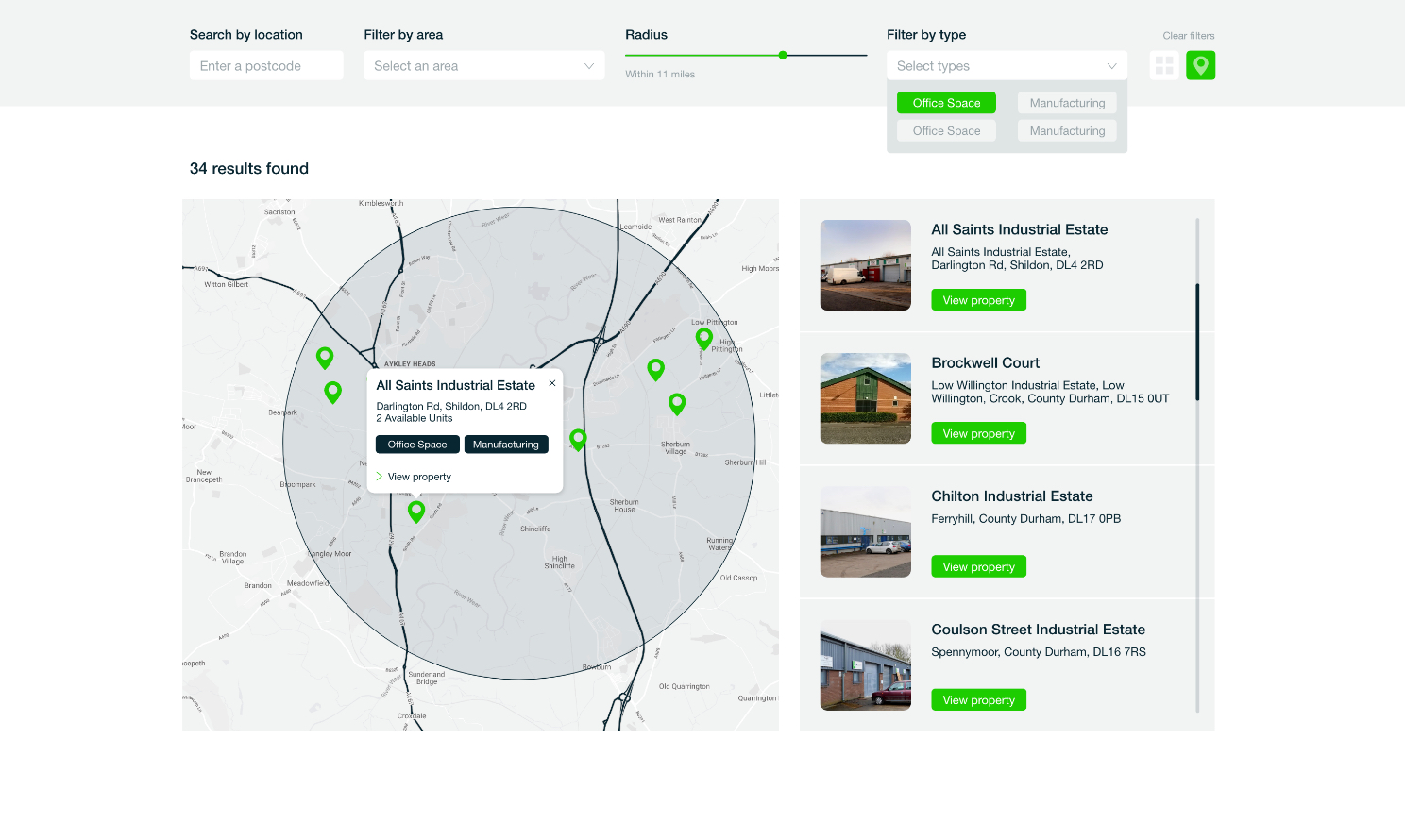The image pertains to a real estate search interface. At the top, there's an option to search for a location. Users can filter results by area, apply a radius filter, or refine their search by type. On the left side, a sidebar displays that 34 results have been found based on the user's query. The main section features a map with a region shaded in dark gray, representing the search results area, while the surrounding regions are in light gray. The map is detailed with roads and town names, making it easy to navigate. Prominently featured locations include All Saints Industrial Estate, Brockwell Court, Clifton Industrial Estate, and Cauldron Street Industrial Estate. The highlighted All Saints Industrial Estate indicates its specific location on the map. This website aids users in narrowing down their desired locations, providing clickable points for further research on potential opportunities, and ultimately helping users decide the best area to settle in based on their preferences.